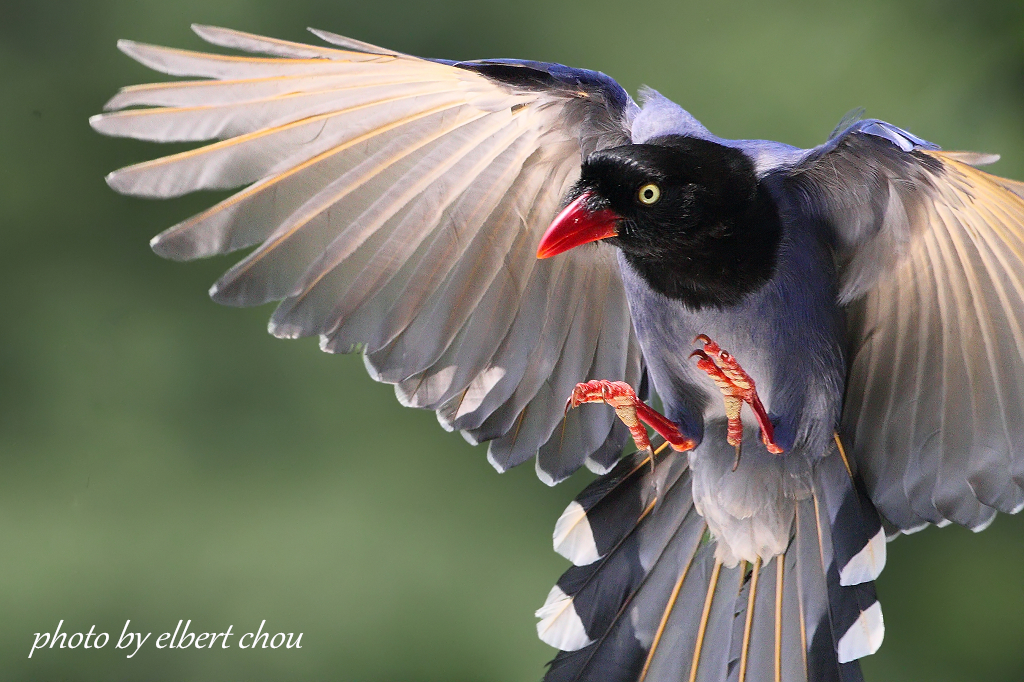This photograph, credited to Ebert Chu, captures a strikingly vibrant bird mid-flight against a blurred, olive-green background. The bird, which appears to be in the process of landing, is predominantly blue with a distinct black head, a vivid red beak, and matching red feet. Its wings are majestically outstretched, revealing a contrast of blue feathers on top and white underneath. The bird’s round yellow eyes, with sharp black pupils, are wide with an expression of fear. Its claws are outstretched, as if ready to grasp a branch that remains out of sight. The image is detailed enough to see the bird's underbelly as it approaches the landing, making for an intense and dynamic visual.